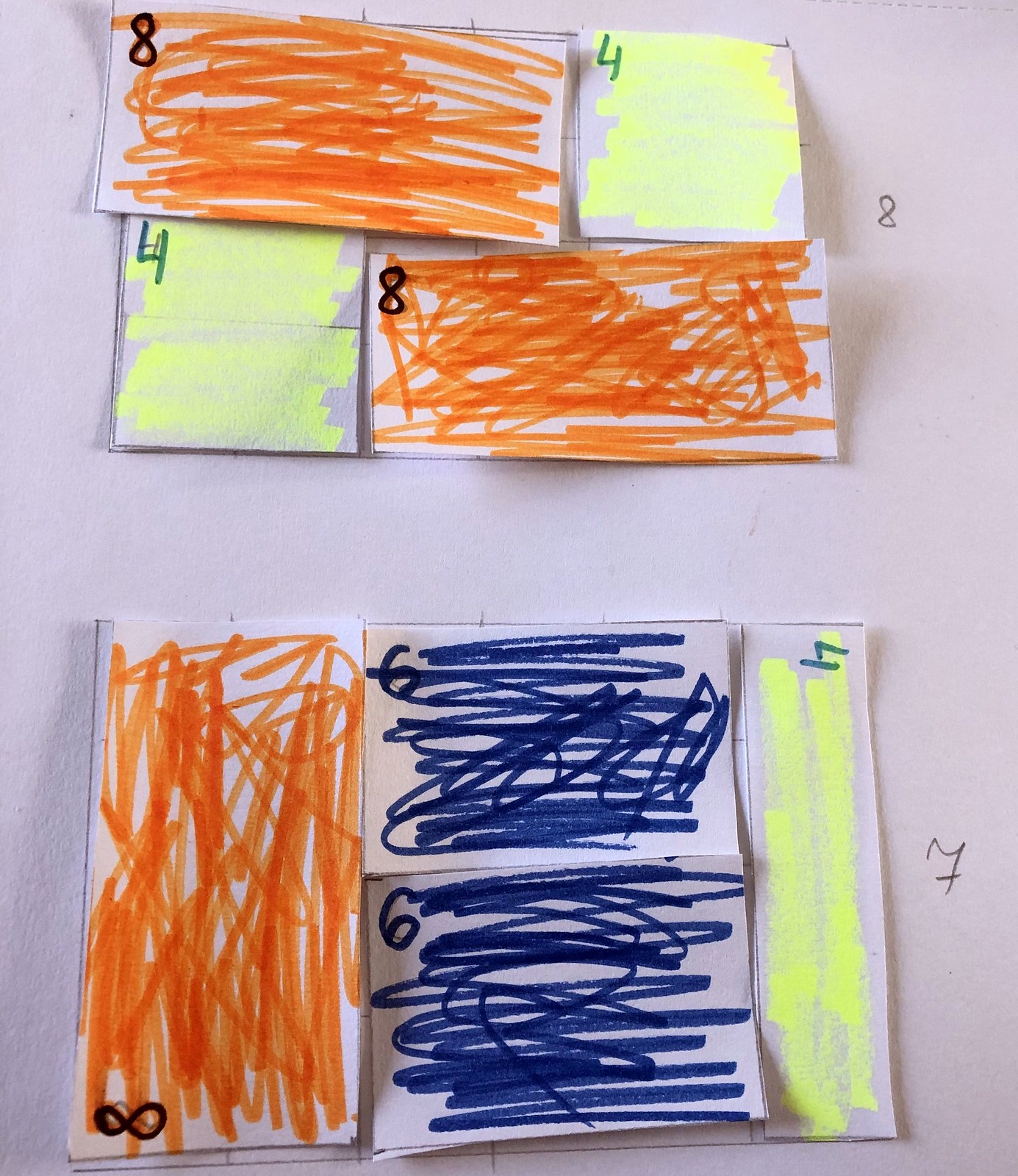The image consists of two vertically stacked pictures, each with a white background, displaying various colored, folded, and cut pieces of paper.

**Top Image:**
1. **Upper Row**:
   - On the left, about an inch from the edge, there's a horizontally oriented rectangular envelope, shaded orange with back-and-forth strokes. It features a black number eight in the top right corner.
   - To the left of this envelope, there's a small, square piece of paper shaded lightly with a yellow highlighter, also with back-and-forth strokes, and a black number four in the top left corner.
2. **Lower Row**:
   - On the left, a small square, colored similarly with a yellow highlighter, has a green number four in one corner.
   - To the right, there's a longer rectangular piece shaded orange with a black number eight in the corner.
   - Positioned almost between the yellow square with the green four and the orange rectangle with the black eight, there is another black number eight.

**Bottom Image:**
- Oriented vertically, this image also features a white background.
1. **Left Side**:
   - A long rectangular envelope shaded orange with vertical back-and-forth strokes. A black number eight is in the bottom left corner.
2. **Middle**:
   - Two vertically stacked rectangular envelopes, both shaded blue:
     - The top one has a black number six in the top left corner.
     - The bottom one is identical to the top.
3. **Right Side**:
   - A long, narrow rectangular piece, about half the width of the orange envelope, shaded in yellow. It has a green number four in the top right corner, with the four positioned sideways (rotated such that the bottom of the number faces left). Just outside of this piece, there's a black number seven.